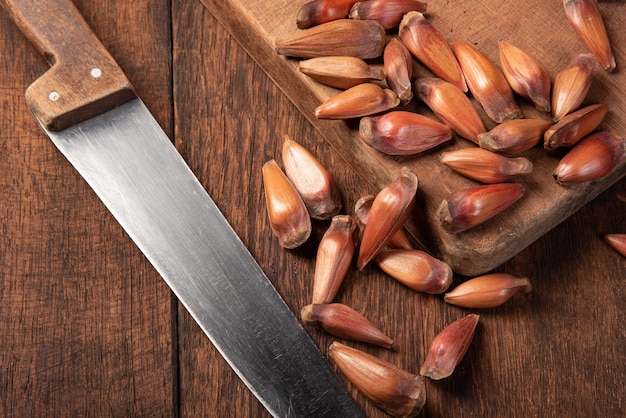In this close-up image, a longer, older knife with a brown wooden handle is situated to the left, while the blade, adorned with white lines and a shiny appearance, partially enters the frame. To the right of the knife, a cutting board occupies the scene's bottom left-hand corner, set atop a dark oak-patterned table that bears evidence of previous cut marks. Scattered across and near the cutting board are approximately a dozen reddish-brown nuts, some of which have spilled onto the table. These nuts, which vary in shades from light green to dark brown, are shiny and exhibit a smooth white interior where some have been broken or cut. The composition suggests a moment halted in food preparation, capturing the contrasting textures and hues of the knife, nuts, and wooden surfaces.